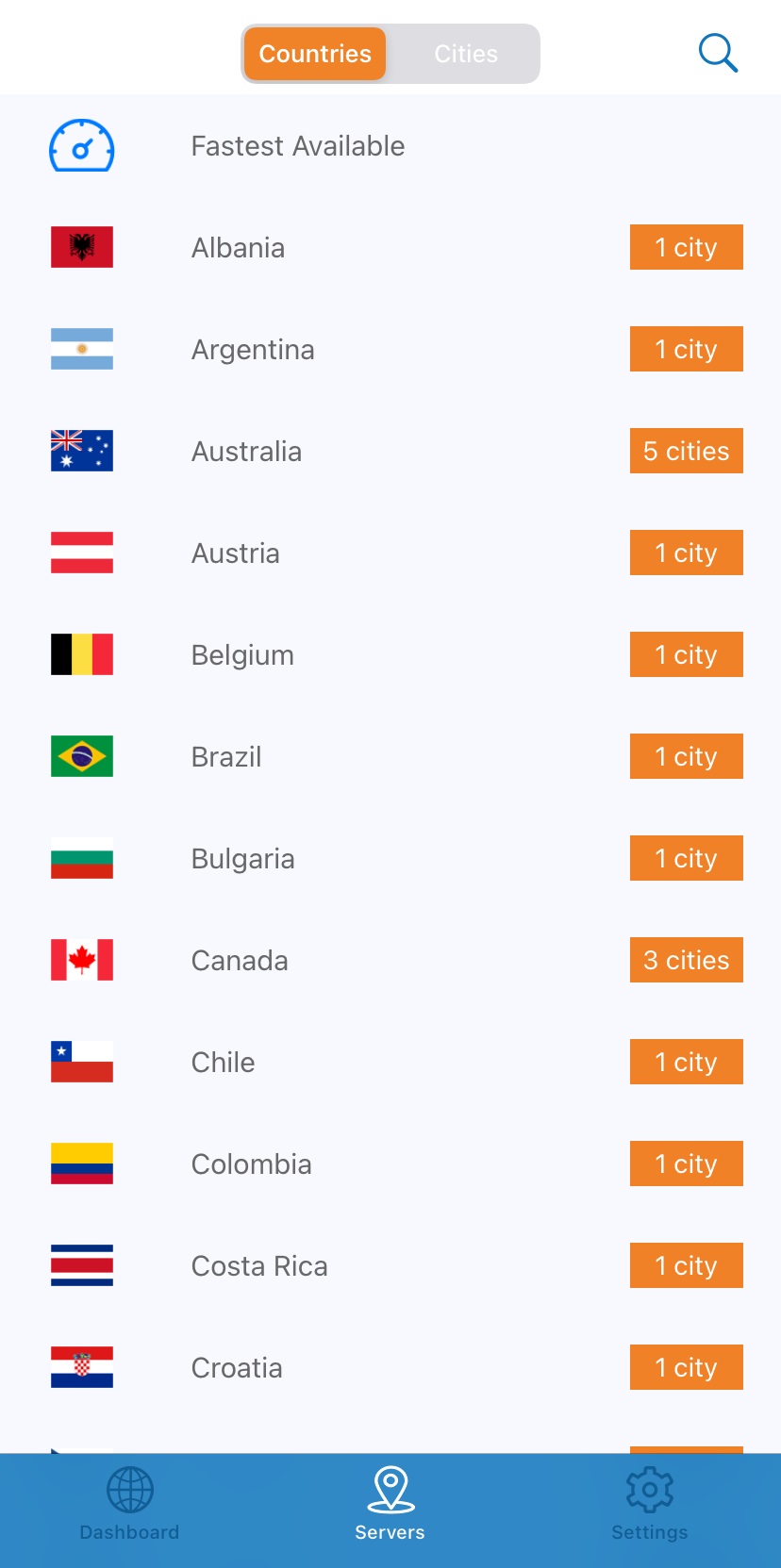The image features a light blue background with an interface related to country and city selection. At the top of the interface are two buttons—a vibrant orange button labeled "Countries" and a light gray button labeled "Cities." Adjacent to these buttons is a small blue magnifying glass icon, presumably a search function.

Beneath these elements, the text "Fastest Available" is displayed prominently on the blue background. Below this, there is a list of countries, each accompanied by an orange button and a flag. The list includes:

- Albania with an orange button labeled "1 city"
- Argentina with an orange button labeled "1 city"
- Australia with an orange button labeled "5 cities"
- Austria with an orange button labeled "1 city"
- Belgium with an orange button labeled "1 city"
- Brazil with an orange button labeled "1 city"
- Bulgaria with an orange button labeled "1 city"
- Canada with an orange button labeled "3 cities"
- Chile with an orange button labeled "1 city"
- Colombia with an orange button labeled "1 city"
- Costa Rica with an orange button labeled "1 city"
- Croatia with an orange button labeled "1 city"

Part of the list is cut off at the bottom of the image. In the lower section, there is a blue box containing options like "Dashboard," "Servers," and "Settings."